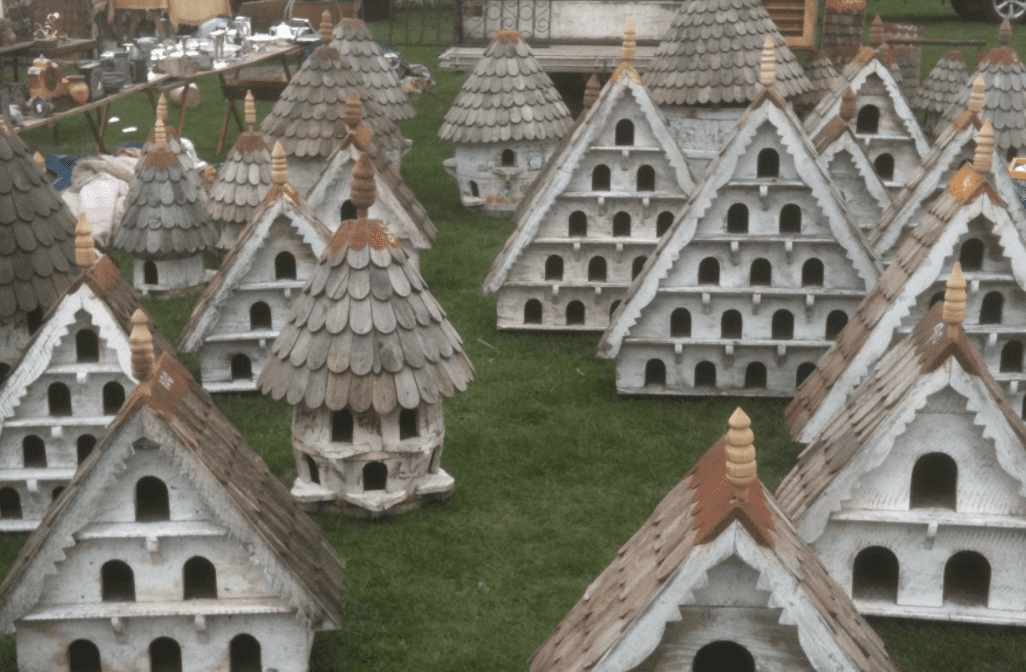The photograph captures a collection of birdhouses displayed on lush green grass, possibly indicative of a yard sale or an outdoor showcasing. The sky appears cloudy, contributing to the serene atmosphere. A notable centerpiece is a group of birdhouses, predominantly white with dark, wooden shingled roofs that resemble small brown ovals. These birdhouses vary in design but are mostly triangular, with the roofs extending down to the ground to form an A-line shape. They feature multiple levels of oval-shaped entryways, arranged from one at the top to five at the bottom. An estimated eight or nine of these birdhouses stand out among the approximately 15 to 20 displayed, each uniquely adorned with tiny windows and door cutouts. In the background, there's an assortment of tables displaying glassware and other items, further enhancing the scene's charm.